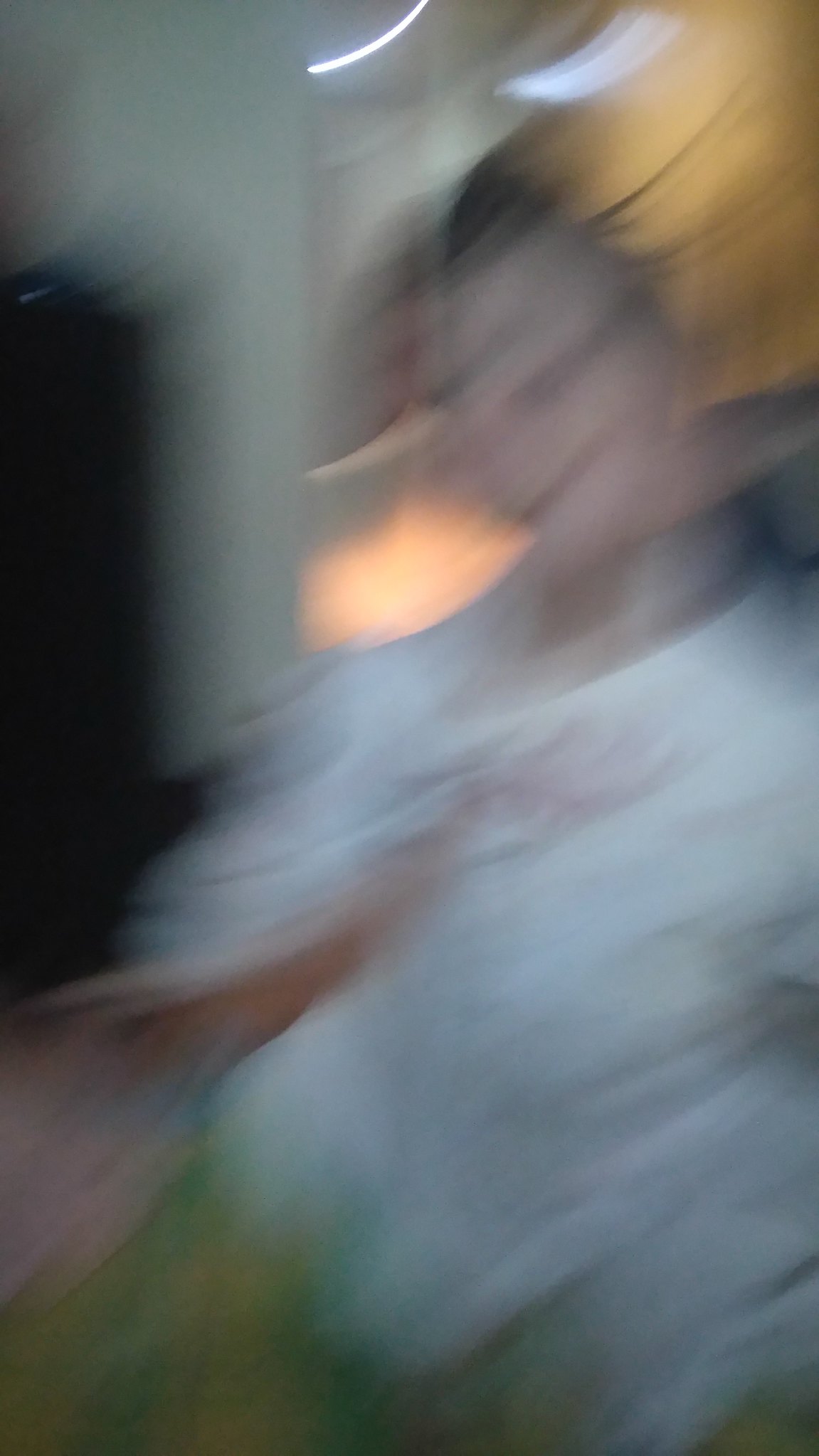This photograph captures a dynamic, blurry image of a woman in motion, likely achieved through a combination of out-of-focus settings and time-lapse exposure. She appears to be dancing gracefully in a flowing white dress. The backdrop consists of a green rug laid over a pink floor, adding a burst of vividness to the scene. In the background, white walls enclose the room, contrasted by a dark-colored door. There is also a light source illuminating part of a wooden wall behind her. Due to the unique shutter speed, the woman's face and body are captured in a series of overlapping images, creating a surreal blend of her motions over several moments, with her mouth appearing as a streak due to her movements during the exposure. The overall effect is a visually intriguing representation of movement and light.